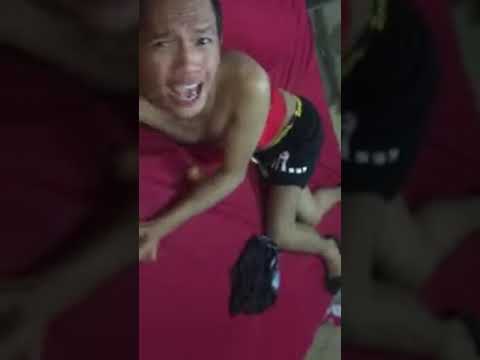The photograph captures a distressed person, potentially of Asian descent, lying on a red or purple mattress or possibly a futon. The image is divided into two parts: the background is zoomed in and obscured with a darker filter, while a spliced-in central portion reveals the same scene zoomed out. The individual, positioned centrally, is wearing a red tube top, a black mini skirt or shorts, and black heels. Their expression conveys terror or anger, with wide-open eyes and mouth, clearly not comfortable or happy. The scene also includes additional clothing items and what appears to be a purse on the bed. The overall composition is framed on the sides with black rectangles, enhancing the eerie, candid nature of the photograph. No explanatory text accompanies the image.